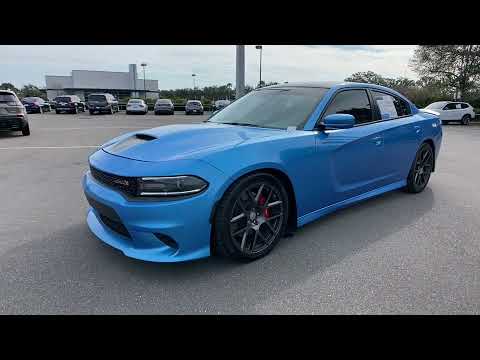This color photograph, taken in landscape orientation, depicts a light blue four-door sedan, likely a Dodge Charger, parked in a car dealership lot. The image is framed by a black bar at the top and bottom. The car, positioned at an angle, faces the left side of the photo, allowing a clear view of its left front headlight but obscuring the right front light and both taillights. A white sticker in the rear windshield provides details about the car, reinforcing its status as a vehicle for sale. The background reveals a variety of parked cars, including SUVs and other sedans, suggesting a mix of models possibly available for viewing. Beyond the vehicles, a gray dealership building and a cloudy blue sky are visible. Sparse trees can be seen in the upper right section of the image, and a slight shadow is cast by the featured car, enhancing the scene’s depth and realism.